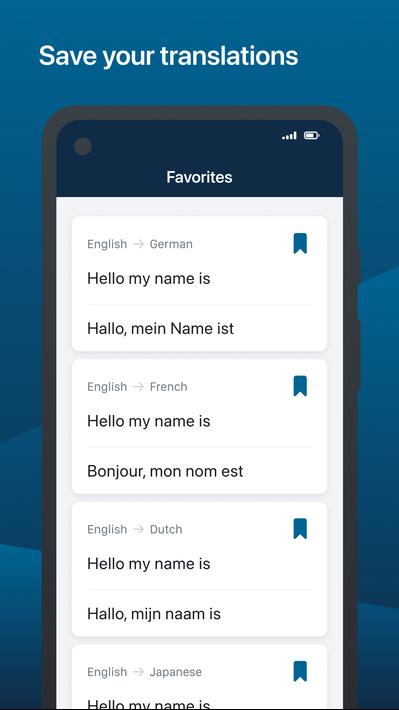The image depicts a screenshot of a translation app displayed on a cell phone. In the top left corner of the screen, there is a gray-shaded text box labeled "Flag as inappropriate." The background of the screen is primarily blue, featuring white text that reads "Save your translations." 

Central to the screen is a navy blue category box titled "Favorites." Below this, the content is organized line by line, showing translations from English to several languages. The phrases read:

1. English to German: "Hello, my name is" (translated as "Hallo, mein Name ist")
2. English to French: "Hello, my name is" (translated as "Bonjour, mon nom est")
3. English to Dutch: "Hello, my name is" (translated as "Hallo, mijn naam is")
4. English to Japanese: "Hello, my name is" (translation appears incomplete as nothing follows)

To the right of each translation, there are bluish-green icons indicating these options are clickable. None of the icons appear to be selected, suggesting no translation has been saved as a favorite yet. The overall layout and design strongly suggest this is a functional translation app user interface on a mobile device.